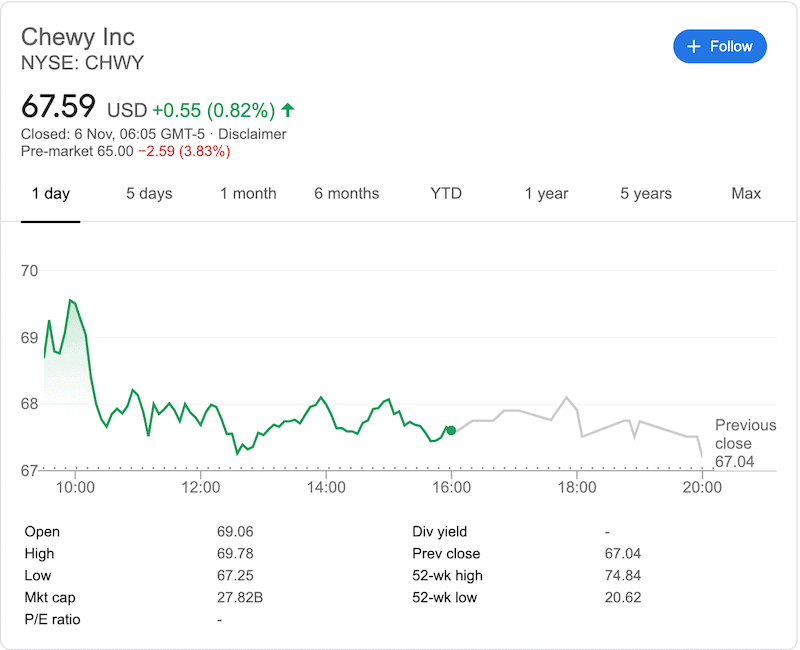The image displays a detailed stock reading for Chewy Incorporated (NYSE: CHWY). In the top left corner, the company name and ticker symbol are prominently featured. On the top right, there's a blue oval button labeled "Follow" with a plus sign. The current stock price is shown as $67.59 USD, with a positive change of $0.55 (0.82%) indicated in green and an upward arrow.

Below this information is a line graph illustrating the stock's performance across various time frames: one day, five days, one month, six months, year-to-date, one year, and five years. The graph line is green from one day to year-to-date, and gray from year-to-date onwards, suggesting a decline in stock value. A horizontal axis at the bottom of the graph indicates time.

Further details are provided beneath the graph, including:
- Opening price: $69.06
- Day's high: $69.78
- Day's low: $67.25
- Market cap: $27.82 billion
- P/E ratio: Not available
- Dividend yield: Not available
- Previous close: $67.04
- 52-week high: $74.84
- 52-week low: $20.62